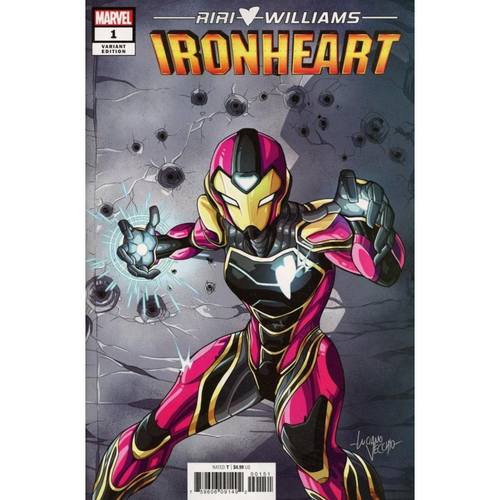The image depicts the front cover of Marvel's comic book, Issue #1. In the top left corner, the classic red Marvel logo stands prominently with the indication that this is a variant cover, suggesting multiple cover designs exist for this issue. The comic introduces "Ironheart," the female counterpart of Iron Man. The character's name, "Riri Williams," is featured at the top in white letters, separated by a heart symbol to creatively denote Ironheart. The signature at the lower right corner of the cover is presumably that of the artist, albeit not clearly legible.

Ironheart's armor, tailored for a female physique, incorporates slightly darker crimson tones compared to Iron Man's traditional red, along with gold and black accents. Notably, she sports a black breastplate in place of Iron Man's iconic chest reactor. Her costume also includes glowing palms. Ironheart is depicted striking a combat-ready pose against a gray, battle-worn wall, peppered with ammunition rounds. The artwork follows a manga-inspired style, emphasizing the character's slim waist and prominent hips. Below the central image, barcode UPC coding is visibly positioned, aligning with commercial distribution practices.